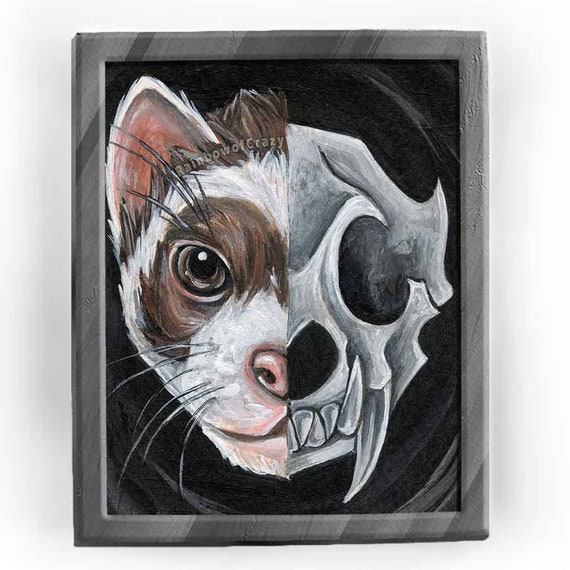This artwork features a striking dual-sided depiction, framed in a thin gray frame, set against a swirling black background. The left half portrays a cat-like creature, featuring a pink ear, a white muzzle, and a brown and white fur pattern with a distinctive patch around its eye. The left side of its face also includes delicate white whiskers and long eyelashes. Contrasting sharply, the right half presents the skull of the same creature, highlighted in white and light gray tones, showcasing menacing fangs and larger teeth, starkly emphasizing the skeletal structure. The meticulous division of the face provides a captivating juxtaposition of life and death within a unified form.